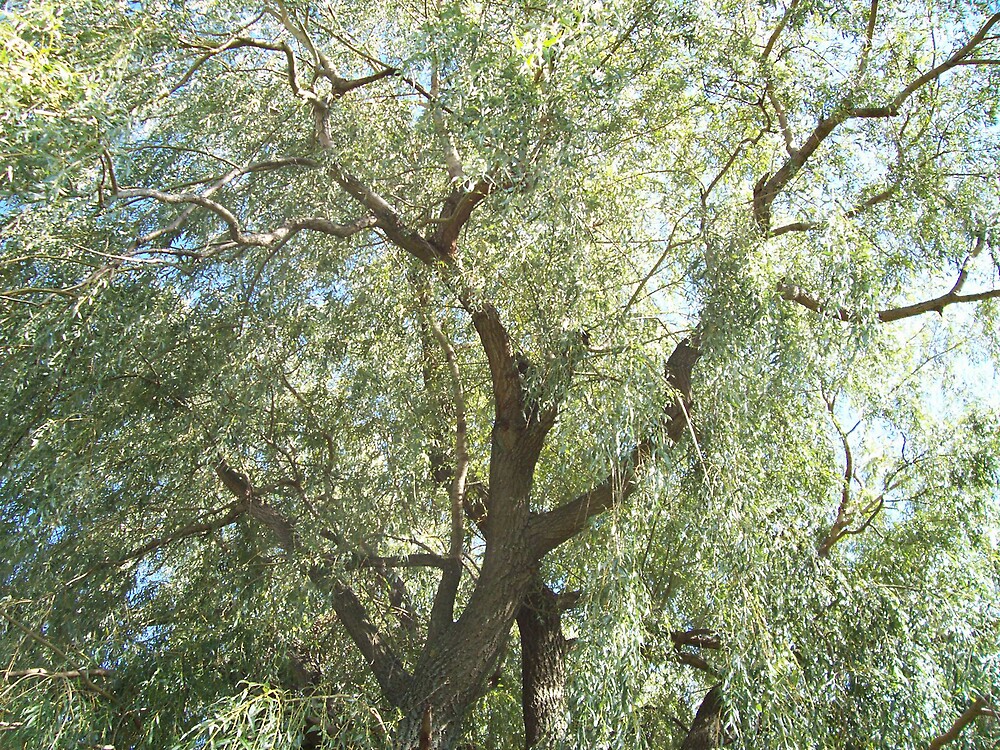This image captures a dense and flourishing green canopy of leaves and branches, suggesting either one large tree or possibly multiple trees, with some debate about the exact number. Dominating the scene is a vibrant mix of light green foliage, interspersed with leaves showing shades of yellow and green, and hinting at some orange-gray hues, indicating parts that might be dying. The tree trunks and branches start from the bottom but their bases are not visible in the frame. Thick branches give rise to thinner offshoots, creating an intricate network of woody stems. The sky provides a transitioning backdrop of light to darker blue, adorned with patches of white clouds peeking through the verdant foliage. The overall setting is rich with natural elements, and the contrasting blue sky emphasizes the lush, thriving, yet somewhat deteriorating tree leaves and branches.